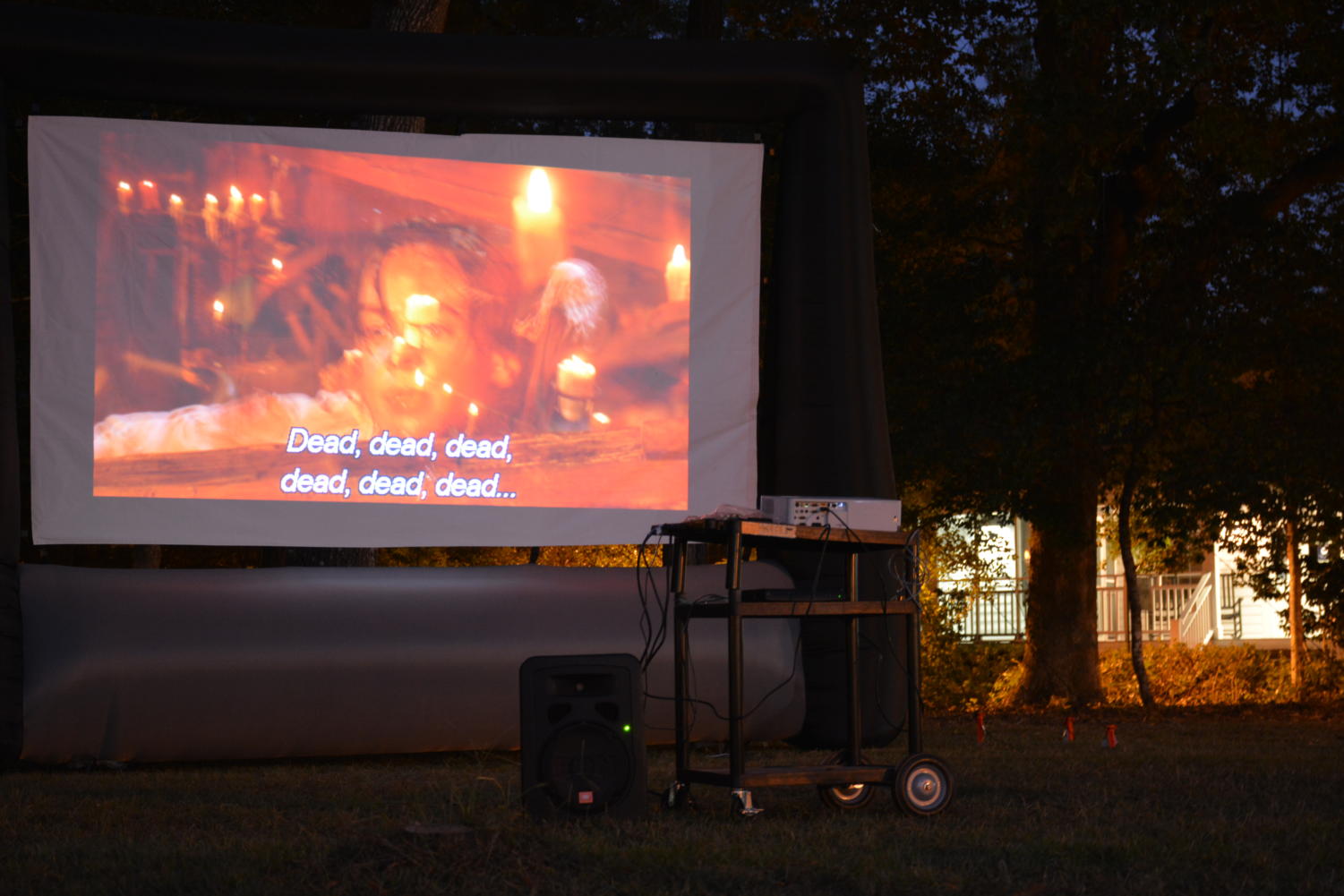The photo captures an impromptu backyard movie screening, featuring a large inflatable projector screen taking up two-thirds of the left side of the image. A white projector, placed atop a compact rolly table with four wheels, projects a movie onto the screen. The scene depicted on the screen is bathed in a red glow, showing a woman with subtitles repetitively displaying the word "dead" six times. Adjacent to the projector on the grass is a substantial speaker, with a noticeable green light indicating it is powered on. The right one-third of the photo reveals more of the yard, including a large tree and a house in the background. The setting hints at an outside cinema ambiance with the added detail of a mysterious, almost ritualistic feel, complemented by the presence of a house and possibly an office or classroom space in the distance.